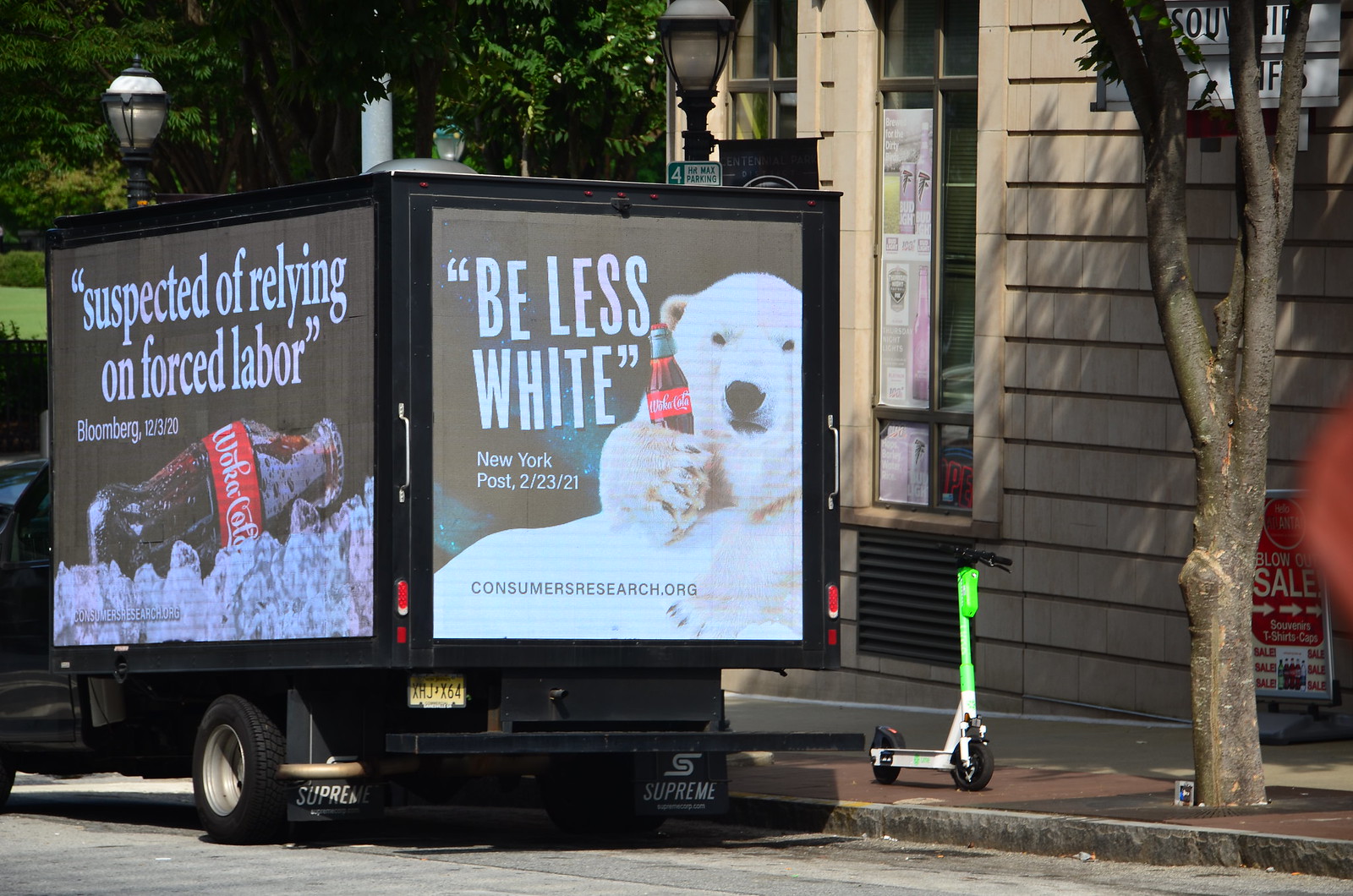A box truck is parked near the curb on a street, close to a building with a tree beside it. A lime scooter is stationed between the truck and the tree. The side of the truck features an advertisement displaying a bottle of Coca-Cola lying on a bed of ice, with the text above it stating, "Suspected of Relying on Forced Labor." This text references Bloomberg, dated 10-3-20. On the back of the truck, there is another sign with an image of a polar bear holding a Coca-Cola bottle. Next to the bear, the text reads, "Be Less White," attributed to the New York Post from 2-23-21, with the source ConsumerResearch.org mentioned below. The truck has a door with a handle at the back that suggests possible entry into the vehicle. The street appears relatively empty and features street lamps, with stores visible behind the truck.